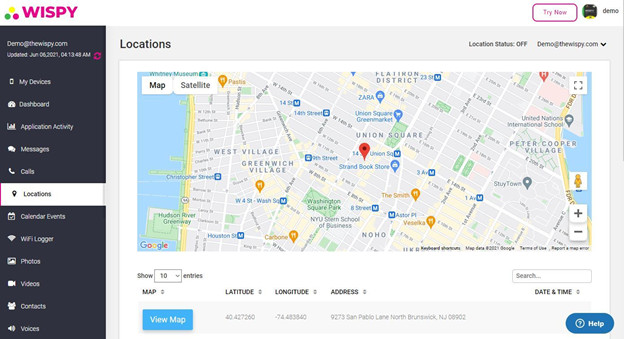**Detailed Caption:**

A detailed screenshot of a location-based service website, titled "Wispy," is displayed. The top-left corner of the interface features the website's title, "Wispy," followed by a contact email, "demo@thewispy.com," and an update timestamp, "Updated June 6, 2021 at 4:13:48 AM." 

The left sidebar contains a variety of navigation sections including: "My Devices," "Dashboard," "Application," "Activity," "Messages," "Calls," "Locations," "Calendar Events," "WiFi Logger," "Photos," "Videos," "Contacts," and "Voices."

On the right side of the screen, there is a map highlighting several notable areas within New York City including West Village, Peter Cooper Village, Union Square, NYU, and the Stern School of Business. Below the map, there is an option labeled "View Map," along with fields displaying latitude and longitude values. Additionally, a related address in New Jersey is indicated beneath the map.